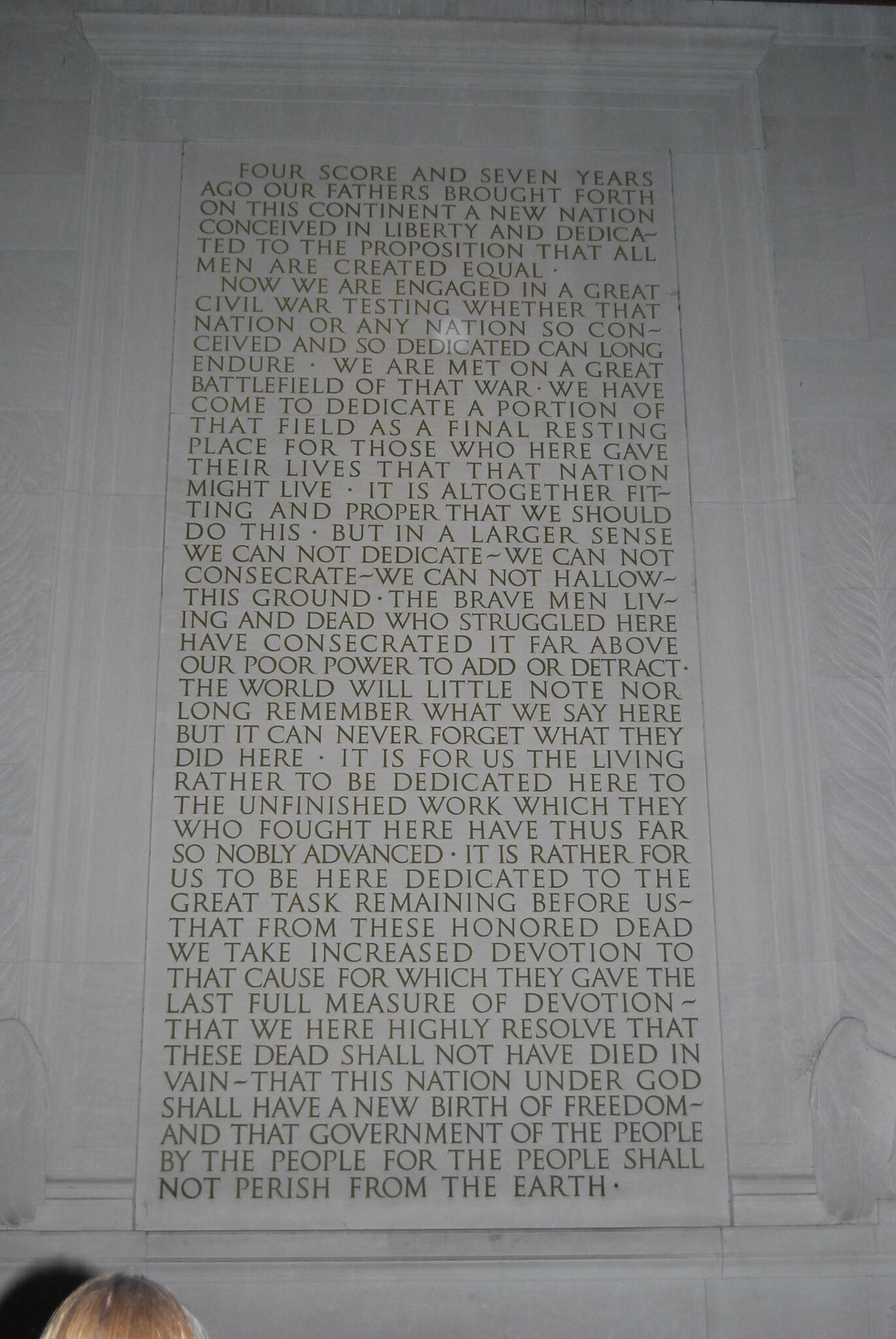The image depicts the Gettysburg Address engraved on a stone wall, viewed from a slightly lower angle, causing the top part of the inscription to be more shadowed. The text, which is framed as if carved within a decorative border, dominates the majority of the image, with the last lines ending towards the lower middle. At the very lower left of the image, the top of a blonde head is visible, along with its shadow cast to the left, indicating perhaps the presence of people visiting this monument. The inscription starts with the iconic words, "Four score and seven years ago our fathers brought forth on this continent a new nation, conceived in Liberty, and dedicated to the proposition that all men are created equal." It progresses through the entire speech, detailing the somber dedication of the battlefield as a resting place for those who sacrificed their lives, the reaffirmation of their cause, and the enduring significance of their actions, concluding with the renowned line, "that government of the people, by the people, for the people, shall not perish from the earth."